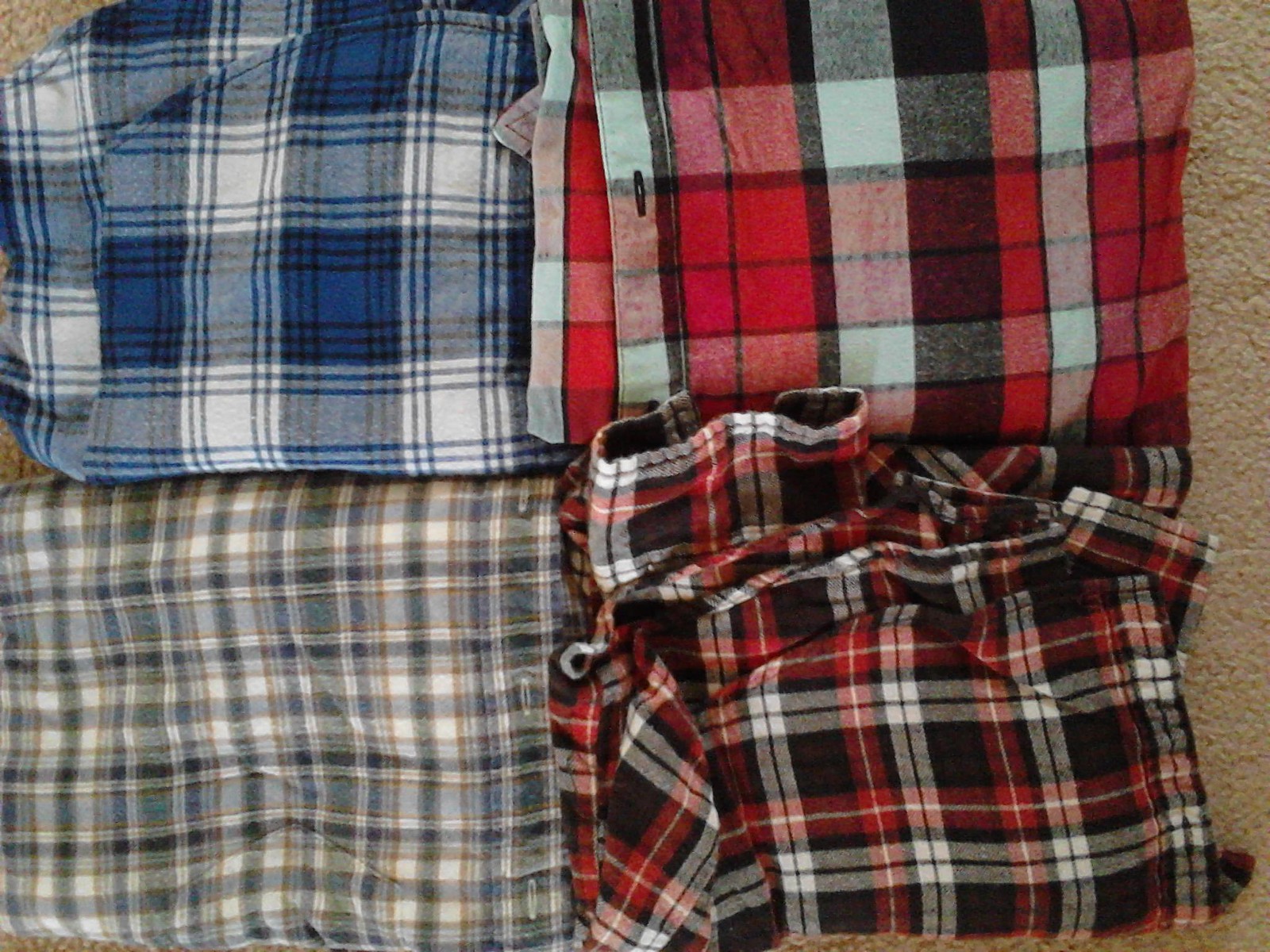This image features a close-up of four neatly folded plaid shirts arranged on a beige carpet, seemingly prepared for sale, perhaps on platforms like eBay or Facebook Marketplace. The shirts are meticulously arranged to showcase the fabric colors, though the fronts and collars are not visible. Starting from the upper left, the shirt is a blue, gray, and white plaid. The upper right shirt displays a gray, white, and red plaid pattern with visible buttonholes. The lower left shirt is adorned with gray, beige, and cream plaid, also showing its buttonholes. Finally, the lower right shirt features a striking white, red, and black plaid design. The overall presentation is orderly and appealing, suggesting a high level of care in the display, ideal for attracting potential buyers.